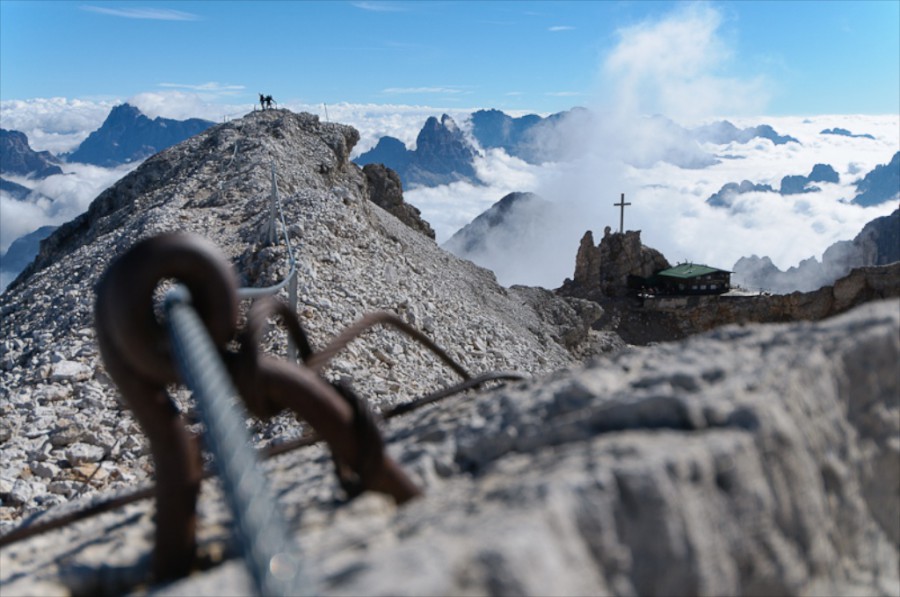The image captures a vibrant outdoor scene set against a mountainous backdrop under a bright blue sky punctuated with white clouds. Dominating the left side of the picture is a sturdy, metallic structure firmly nailed to the ground, with a gray rope threading through a hole in the structure. The rope extends from the foreground, traverses over a hill, and vanishes into the distance, drawing the eye to the horizon. Near the edge of this hill, two individuals appear to be engaged in rock climbing or a similar activity. On the right-hand side, a building with a distinct green roof stands prominently. Behind this building, a large cross rises atop a stone, seemingly perched on a cliff. The scene is flooded with natural light, making colors vivid and details crisp, painting a serene yet dynamic portrait of this mountainous landscape.